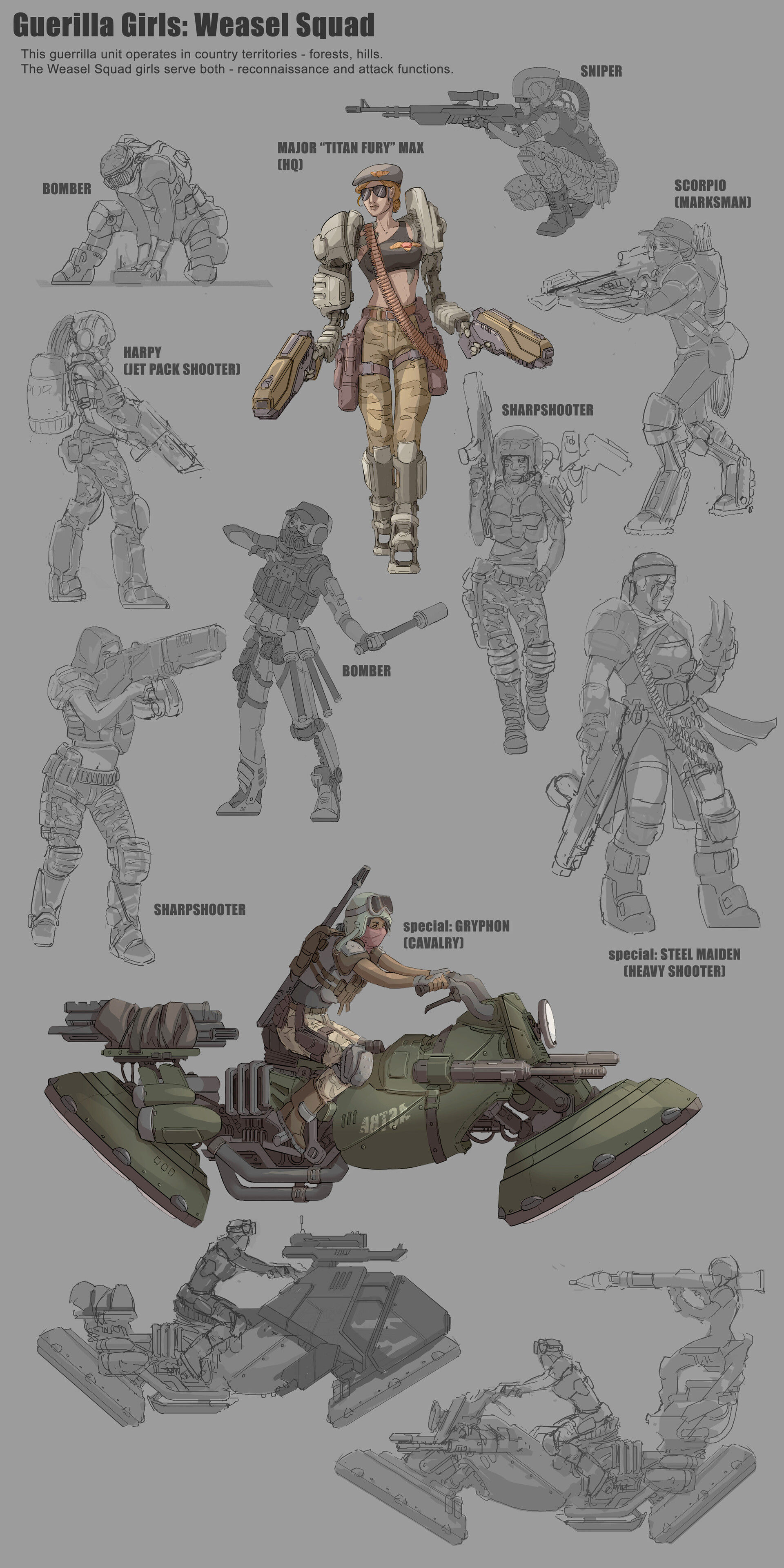This image is a highly detailed poster titled "Guerrilla Girls Weasel Squad," prominently displayed at the top left corner. Beneath the main title, in smaller text, it states, “This guerrilla unit operates in country territories, including forest hills. The Weasel Squad girls serve both reconnaissance and attack functions.” The background of the poster is gray, showcasing a series of sketches and diagrams of the squad members, predominantly in black and white, with some elements in color.

The characters – all women – are depicted wearing military garb, including camouflage pants and a mix of tight-fitting or scantily clad tops. They are heavily armed with large automatic weapons and other artillery. The bottom section of the poster features three women riding hover motorcycles, each labeled with roles such as "Sharpshooter," "Jetpack Shooter," and another "Sharpshooter."

Throughout the poster, various characters are identified with distinct labels and roles, such as "Sniper," "Scorpion," "Marksman," "Major Titan Fury Max HQ," "Bomber," "Harpy," "Special Griffon Cavalry," and "Special Steel Maiden Heavy Shooter." The color palette prominently features greens, camouflage sand, grays, beige, and whites, contributing to the military theme.